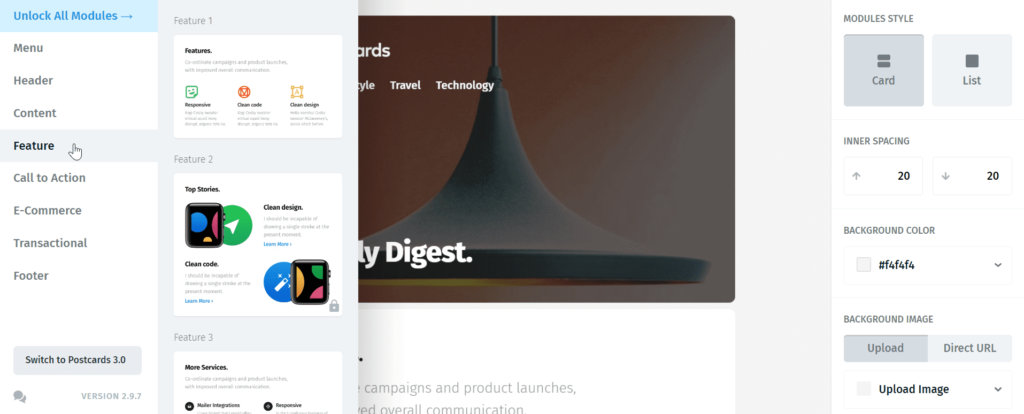The image features a modern hanging pendant light in a rich blue hue. The backdrop of the image is divided into two sections: a dark pink shade occupies the left side, while a bluish-gray shade dominates the right. In the upper left corner of the image, the words "Travel" and "Technology" are displayed prominently, while the word "Digest" stands out in bold white text below these. 

To the far left, there is a blue rectangle containing the phrase "Unlock All Modules" in blue text. Below this heading, a list of choices is available in bold black text, including "Menu," "Header," "Content," "Feature," followed by icons representing actions such as "Call to Action," "E-commerce," "Transactional," and "Footer," possibly indicating clickable links suggested by the presence of a cursor hand icon.

On the right side of the image, there are depictions of cell phones or dark boxes with colorful displays. Above these, the phrase "Top Stories" is written, suggesting featured content or highlights. Adjacent to this section is a distinct blue circle enclosing the image of a white pen, surrounded by three smaller white circles, likely representing a writing or editing function.